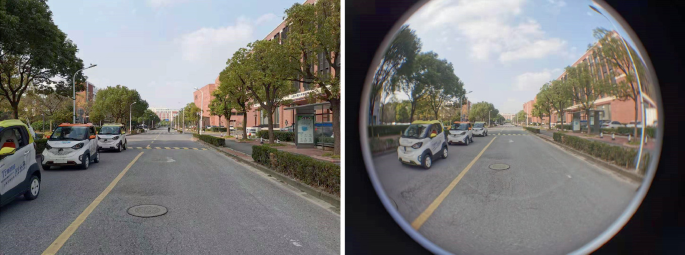The image consists of two photographs of the same street, providing different perspectives. The scene captures a beige or salmon-colored urban backdrop, adorned with trees and a bus stop to the right. Three small cars, potentially electric vehicles, traverse the street divided by a solid yellow line. The left photograph presents a closer, full-on view with the cars appearing nearer, revealing the details of a sewer cover in the foreground. In contrast, the right photograph offers a pulled-back, perhaps fish-eye lens view through a circular frame with a black border, making the cars and surroundings appear slightly distorted and further away. Lush greenery complements the sidewalks, enhancing the meticulously landscaped street, while the familiar traffic and serene ambiance persist across both images.